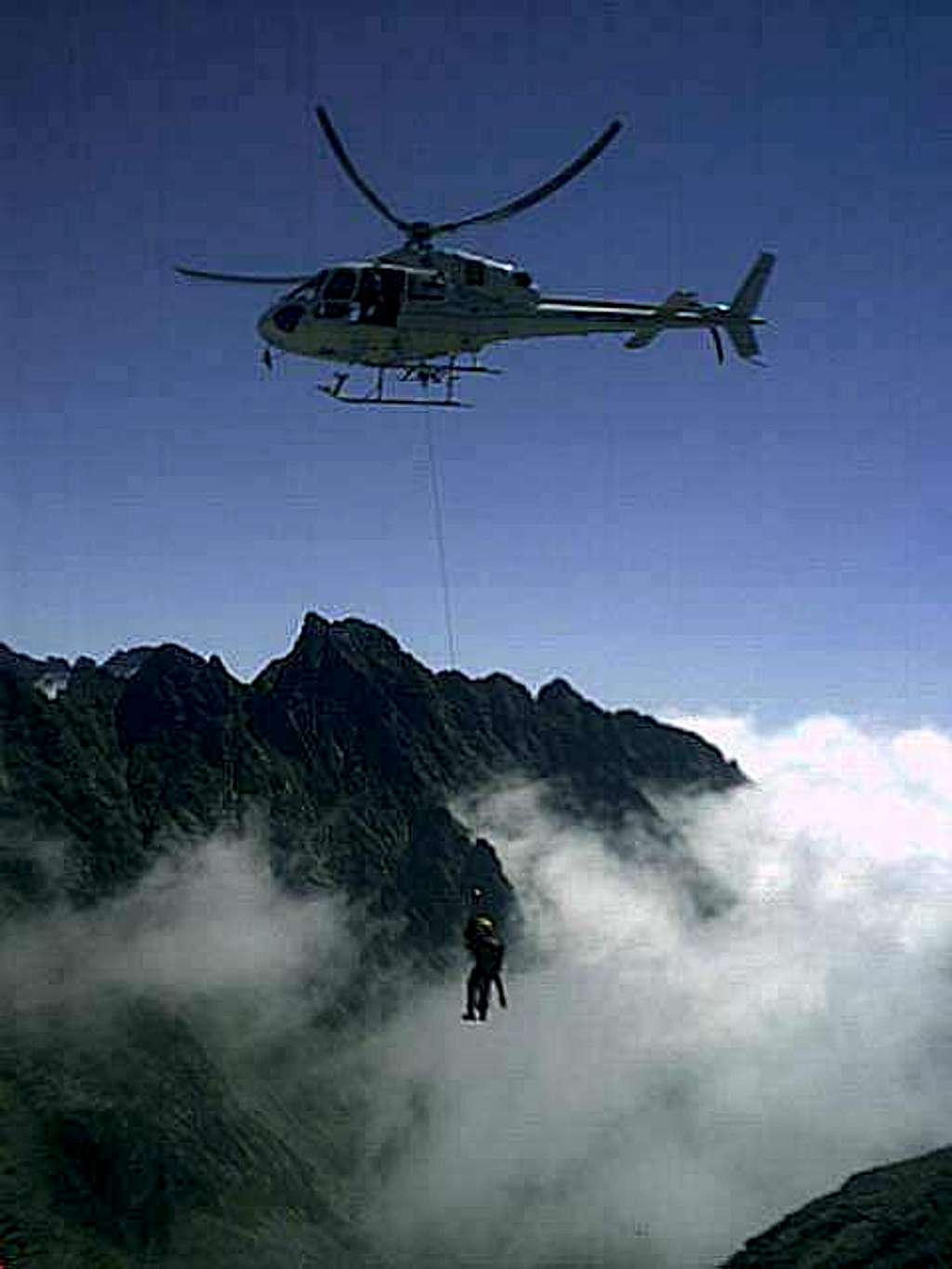The image captures a striking scene of a white helicopter in mid-flight, possibly engaged in a rescue or escort mission. The helicopter, adorned with a blue stripe running from its midsection to the tail, cuts across a vivid blue sky, its main and tail propellers frozen in a blur of motion. Below the aircraft, a man dressed in an all-black outfit with a yellow helmet dangles from a rope, appearing to descend towards the ground. The photo, taken in portrait orientation, prominently features the helicopter in the top center with its nose pointing left. The mountainous backdrop is awe-inspiring, with jagged, dark peaks haloed by misty, fog-like clouds that envelop their bases, offering a dramatic contrast to the crisp, clear skies above. The entire scene and composition suggest both the grandeur of nature and the perilous tasks undertaken by the individuals involved.